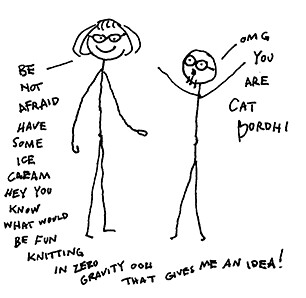This black line drawing on a white background features two stick figures, a man and a woman, depicted with exaggeratedly long arms and legs. The woman, on the left, has short hair curled under her neck, bangs, and is wearing glasses. She is smiling and saying, "Be not afraid, have some ice cream. Hey, you know what would be fun? Knitting in zero gravity. Ooh, that gives me an idea!" A line connects her to the accompanying text. The man on the right has a round head, glasses, and a few chin hairs, hinting at whiskers. He responds with "OMG, you are cat bored." Both figures are positioned vertically and stand next to each other, surrounded by playful, amusing text emphasizing their whimsical conversation.